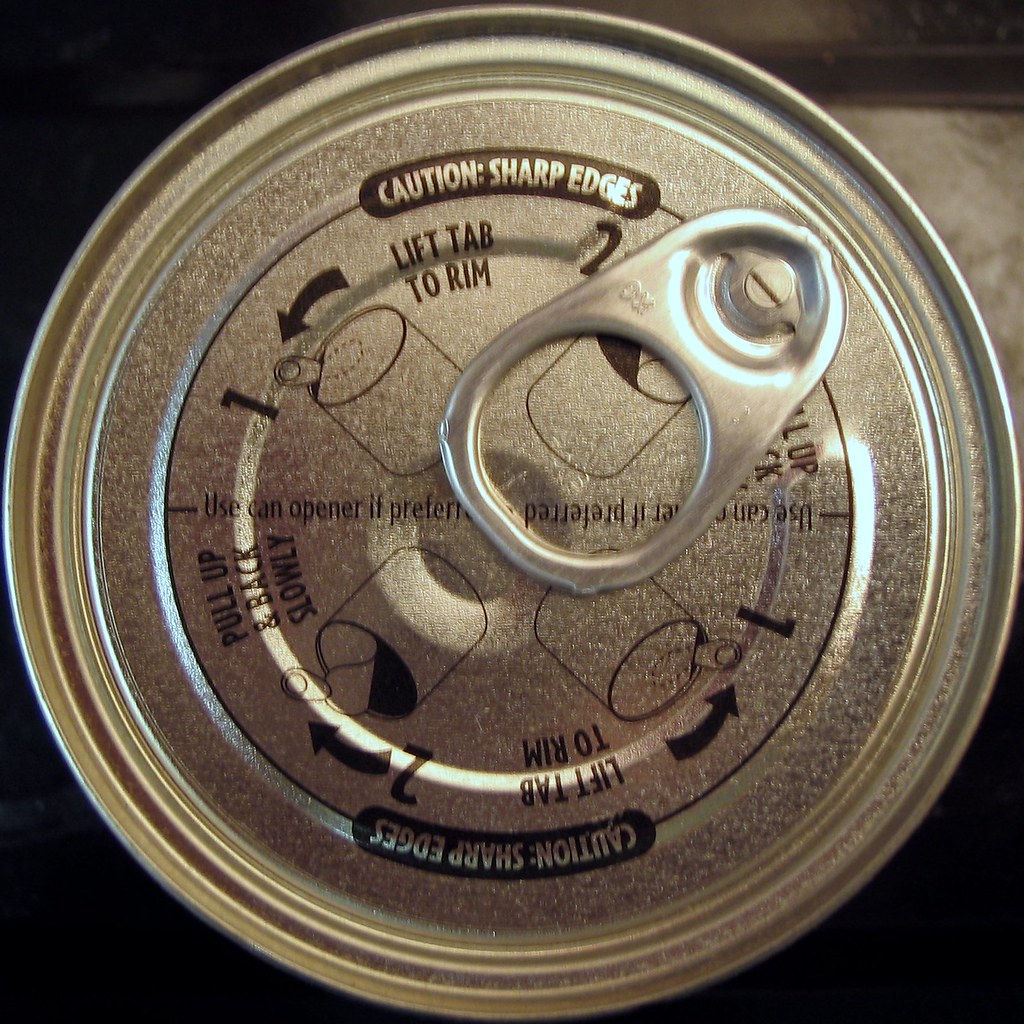This high-resolution, close-up image showcases the top of a sealed can, prominently featuring a pull-tab mechanism. The detailed construction of the pull tab is clearly visible, including the breakaway area and the attachment of the pull ring. The image also captures the instructions for opening the can, which involves lifting the tab to the rim and pulling back slowly to remove the cover entirely, resulting in a full opening rather than just a narrow pour spout. There is a visible warning about the sharp edges that may be present after opening. The background of the image is a dark gray, which contrasts sharply with the metallic sheen of the can top, making the intricate details stand out even more.